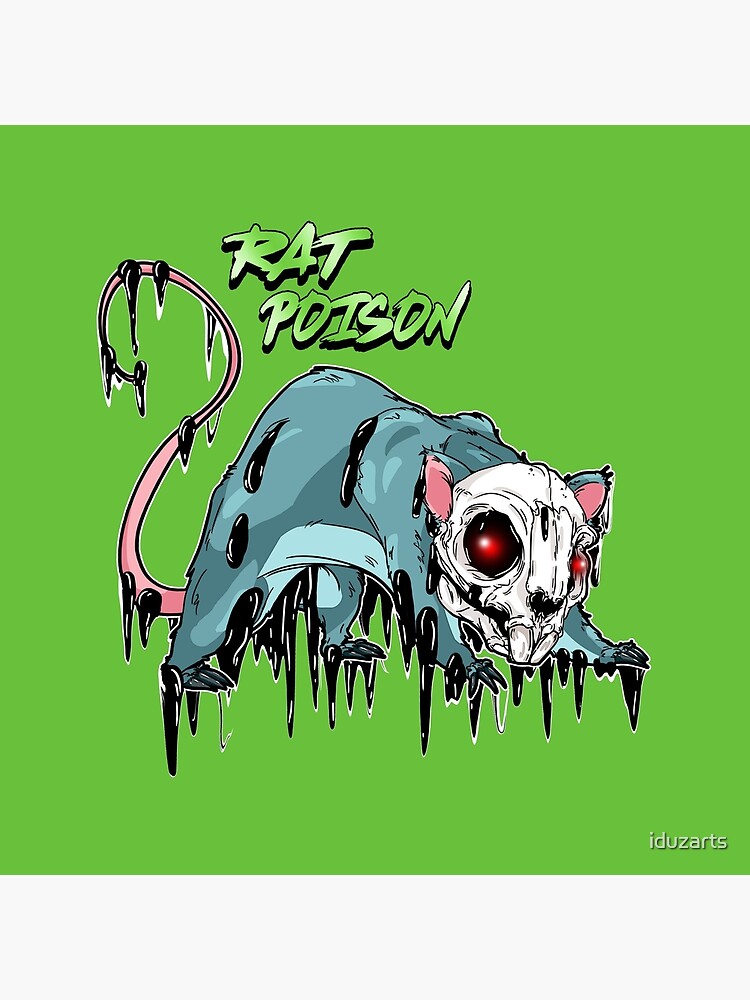This is an artistic sticker or decal with a lime green background. The rectangular image features the text "rat poison" in bold, black outline letters at the center top, in a graffiti-like font. Below the text is a disturbing, cartoon-style depiction of a decaying rat. The head of the rat is a stark white skull, with large, glowing red eyes and two prominent front teeth. The decaying body of the rat is shaded in a grayish-blue color, and it has pink ears and a long pink tail. The rat appears to be in pieces, with areas of its body—including the tail—dripping with a black, gooey, tar-like substance that covers its entire body, especially pooling beneath its feet. This black substance suggests poison, seeping from puncture wounds on its abdomen. The rat's skin looks shriveled and deteriorating. In the bottom right corner of the image, there is a signature in a white font that says "I-D-U-Z-A-R-T-S." The stark contrast between the sickly green background, the black dripping details, and the vivid red eyes contributes to the disturbing and grotesque nature of the illustration.